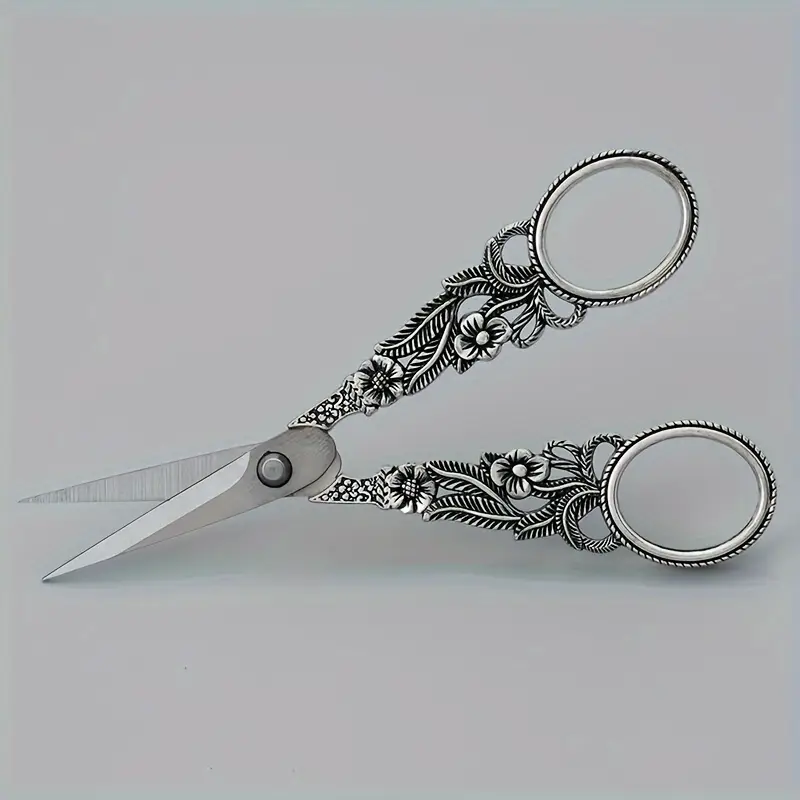This detailed image displays an up-close view of an intricately designed pair of decorative scissors. The scissors are crafted from a silver-like stainless steel with black markings that accentuate their elaborate patterns. The handles feature large oval finger holes, encircled with ornate metalwork. Leading down from the handles, the metalwork transitions into a beautiful floral motif, with long, thin leaves and two flowers on each handle, decorated with black accents to highlight the veins of the leaves and the petals of the flowers. Tiny black dots decorate the flower centers. The floral design is mirrored on both handles and is seamlessly intertwined with additional leaf shapes that form a bow near the top. The cutting blades of the scissors are relatively short, indicating they are likely used for precise, delicate tasks. The entire pair of scissors is displayed against a solid gray background, which enhances their detailed craftsmanship and casts a subtle shadow.